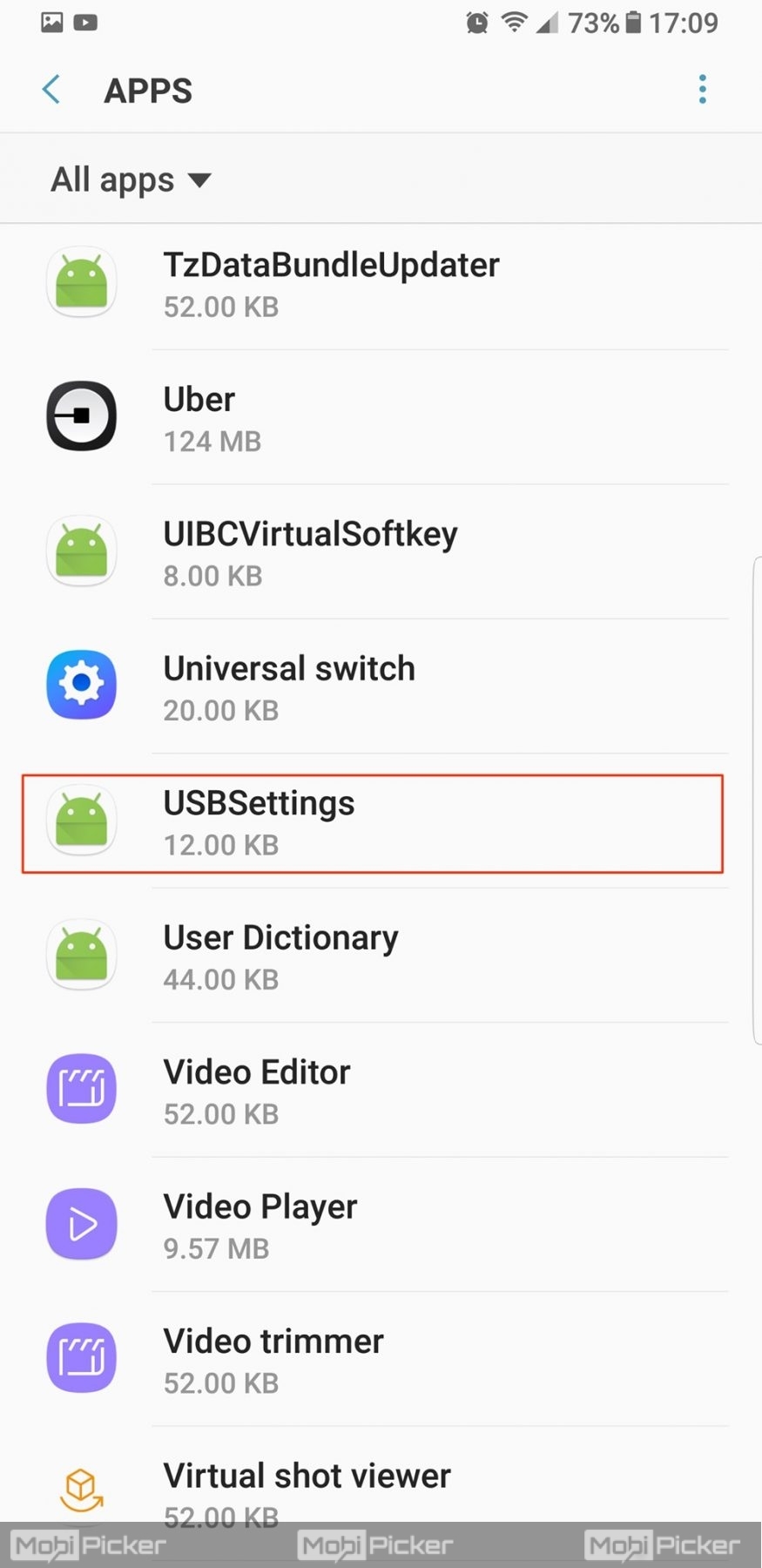A screenshot of a mobile device's storage details is shown with a variety of app data usage statistics. The device's battery is at 73%, and the time displayed is 17:09. The top part of the interface includes an arrow pointing left and three vertical dots indicating additional options. 

The "All Apps" section lists several applications with their respective data sizes:

- **TZ Data Bundle Updater**: 52 KB
- **Uber**: 124 MB
- **UIBC Virtual South Key**: 8 KB
- **Universal Switch**: 20 KB
- **USB Settings**: 12 KB (highlighted with a red rectangle)
- **User Dictionary**: 44 KB
- **Video Editor**: 52 KB
- **Video Player**: 9.57 MB
- **Video Trimmer**: 52 KB
- **Virtual Shot Viewer**: 52 KB

At the bottom of the screen, three instances of "Mobi Picker" are visible in gray text over a light gray rectangular background. This detailed interface showcases the storage usage of various applications, emphasizing the small size of utility apps and the relatively larger size of media-related applications.